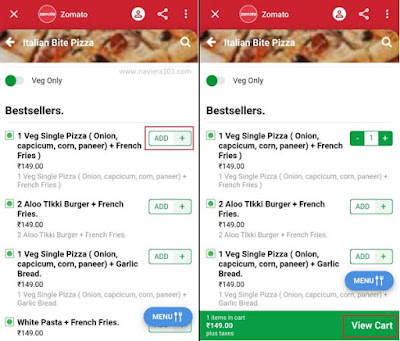This image showcases two different mobile screenshots featuring a food delivery application.

On the left screenshot, the top part is dominated by a large red header. In the upper left corner of the header, there's a white "X" icon. Slightly left of the center of the header is a circular red icon bordered in white, although its white text is too pixelated to decipher. To the right of the circular icon, in bold white lettering, it reads "Zomato." Moving further right within the header, there is a white circle with a red user icon outline, followed by a white share icon, and then three vertical dots indicating a menu.

Beneath the header is a banner displaying a pizza topped with olives, tomatoes, crust, and cheese. Overlaid on the left side of the pizza banner is a bold white arrow pointing left, accompanied by the text "Italian bite pizza" in bold white letters. At the bottom of the banner, a faint gray line acts as a divider, and in small gray font towards the right, it reads "www.naviera101.com."

Further down on the left, there's a toggle option with a green circle on a gray background indicating it is turned off. Next to this toggle, in black text, it says "veg only." Below this, in bold black lettering, it reads "Bestsellers." This section is separated by another faint gray line divider.

The second screenshot, displayed on the right, is not detailed in this description.